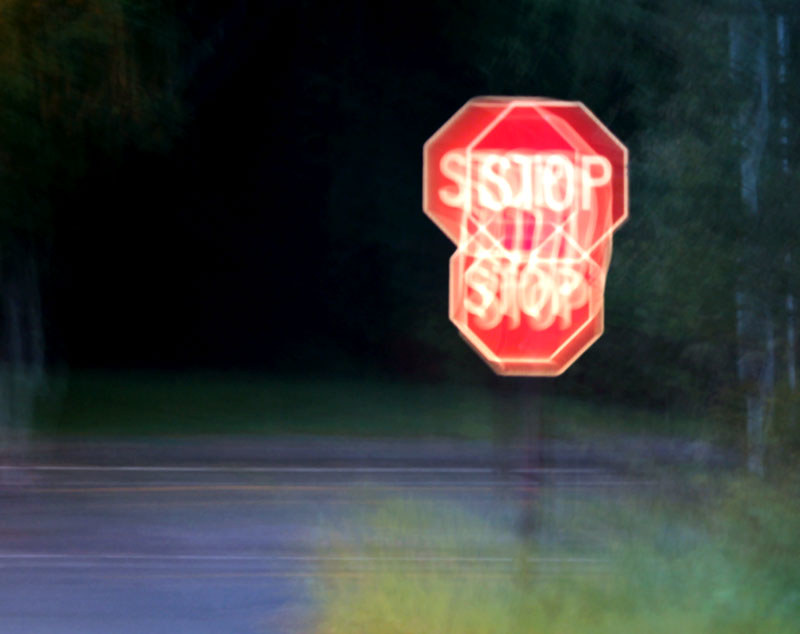The photo captures a blurry nighttime scene outside, depicting a red hexagonal stop sign on a black pole along a grey street with a yellow stripe down the middle. The stop sign, located in the upper middle right of the image, appears several times in overlaid, distorted, and partially transparent layers, creating a ghostly, repetitive effect. The word "STOP" is similarly duplicated and streaked, particularly on the top two and bottom two iterations of the sign. Surrounding the sign are green bushes and tall grass, with the backdrop extending to dark green trees indicating the entrance to a forest. The entire scene is enveloped in a hazy appearance, likely due to camera movement or shaking, which further blurs the bushes, road, and line markings, leaving an eerie and disjointed impression.